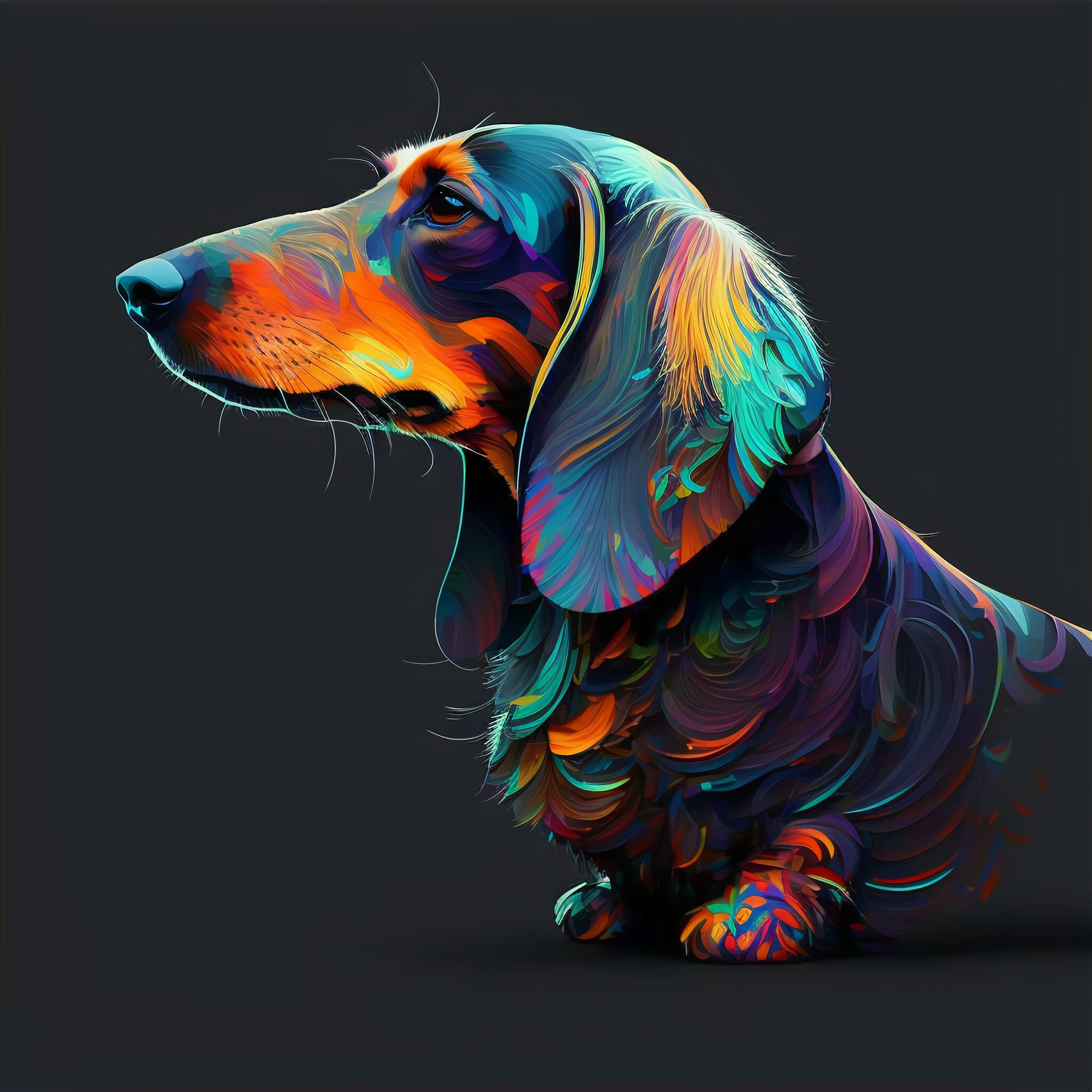The image showcases a computer-generated, colorful portrayal of a dachshund rendered in a psychedelic style. The dog, which has a disproportionately large head and notably short legs, is depicted in profile from its nose to the middle of its back, with only the front two legs visible. The artistic technique used to create the dachshund employs a vibrant palette including shades of orange, yellow, turquoise blue, green, purple, pink, and hints of white whiskers. These colors are applied in swoops, swirls, and random strokes, reminiscent of a graffiti wall mural or piñata design, giving the dog a surreal, almost whimsical appearance. The background is plain and dark, which accentuates the striking, multicolored patterns of the dog's fur. The realistic details, like the whiskers extending from its muzzle and eyebrows, contrast with the abstract coloring, adding depth to the whimsical representation. The dog’s golden eyes and serious expression stand out against the chaotic yet mesmerizing color scheme.